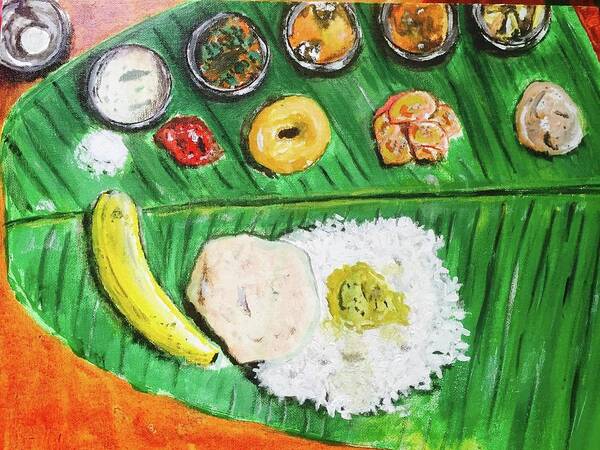The painting portrays a vibrant overhead shot of a large, green serving leaf meticulously arranged with various foods, set against an orange or wooden table backdrop. The leaf, visually prominent with extra lines and a central vein, spans horizontally across the frame. At the top, five round silver bowls line the leaf, containing different colorful substances, perhaps various sauces or salsas: the leftmost bowl holds a white substance, the second bowl has an orange substance with green flecks, the third is light orange, the fourth is a darker orange, and the fifth contains a yellowish-gray item.

Beneath these bowls, a diverse assortment of foods is neatly organized. Starting from the left, there is a white substance presumably linked to the first bowl, followed by a red pepper-like item, a yellow donut or bagel, orange slices, and a congealed brown mass. In the lower half of the leaf, a bright yellow banana or plantain sits on the left, adjacent to a white, pinkish rock-like item atop what appears to be a bed of white rice. Centered on this "rice mat" is a food item with a yellow, mustard-like appearance.

The entire scene is captured with vivid colors and fine detail, emphasizing the leaf's texture and the variety of foods it supports, presenting an inviting, organized display often seen in traditional or cultural food presentations. In the top left corner, a transparent water glass adds a touch of everyday realism to the artistic composition.